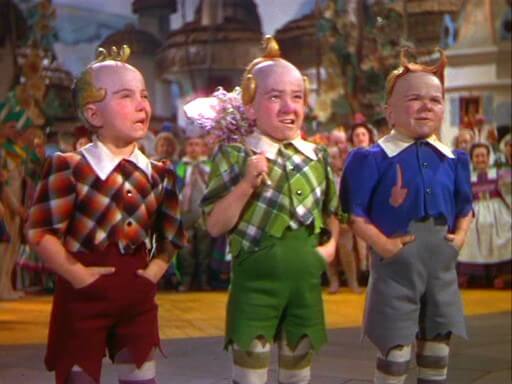The vibrant color photograph captures a scene reminiscent of the original Wizard of Oz movie, featuring three small, gnome-like characters or munchkins in the foreground. These characters, possibly children, are dressed in eclectic and whimsical outfits with distinctively colored and patterned elements. On the left, the character wears a plaid shirt in shades of red, black, and white, paired with red zigzag cut shorts. The character in the middle dons a green, white, and black plaid shirt, green cutoff shorts, and white socks with green stripes. The character on the right sports a blue shirt with a white collar, gray cutoff pants, and white socks with gray stripes. All three characters have golden headpieces, and the one in the blue shirt has a symbol resembling a finger, staff, or wand on the chest area. Behind them, the background reveals a set of old buildings resembling townhomes or factories, as well as a group of figures, including both men and women, adding depth and context to the scene. The characters’ hair is styled into tight curls, creating a notable contrast with their receding hairlines, and each character’s outfit is complemented by large white collars and knee-length shorts. This lively and detailed tableau conjures the iconic and fantastical atmosphere of the classic film.